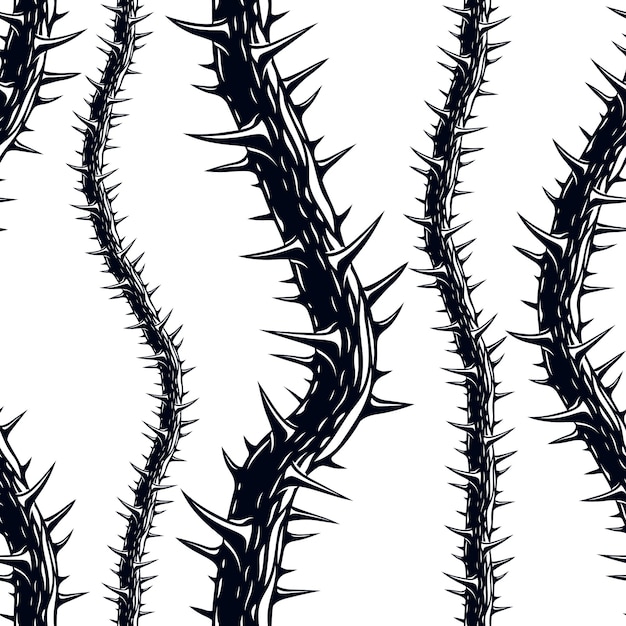The artwork is a black and white drawing of five thorny vines extending from the bottom to the top of the image. Each vine follows a wavering pattern, curving slightly to the right and then back to the left repeatedly. They are evenly spaced with narrow gaps between them, creating a pleasing symmetry. The middle vine is highlighted with the darkest tones and features the largest thorns, making it a focal point. The outer vines, appearing to be slightly out of focus, exhibit fewer thorns compared to the central one. The one on the far right is thicker than the adjacent vine but thinner than the central vine. The leftmost vine occupies the top left and bottom left corners of the image, contributing to the balanced layout. Overall, the distinct yet uniform structure of the vines and their thorny details dominate this intricate artwork.